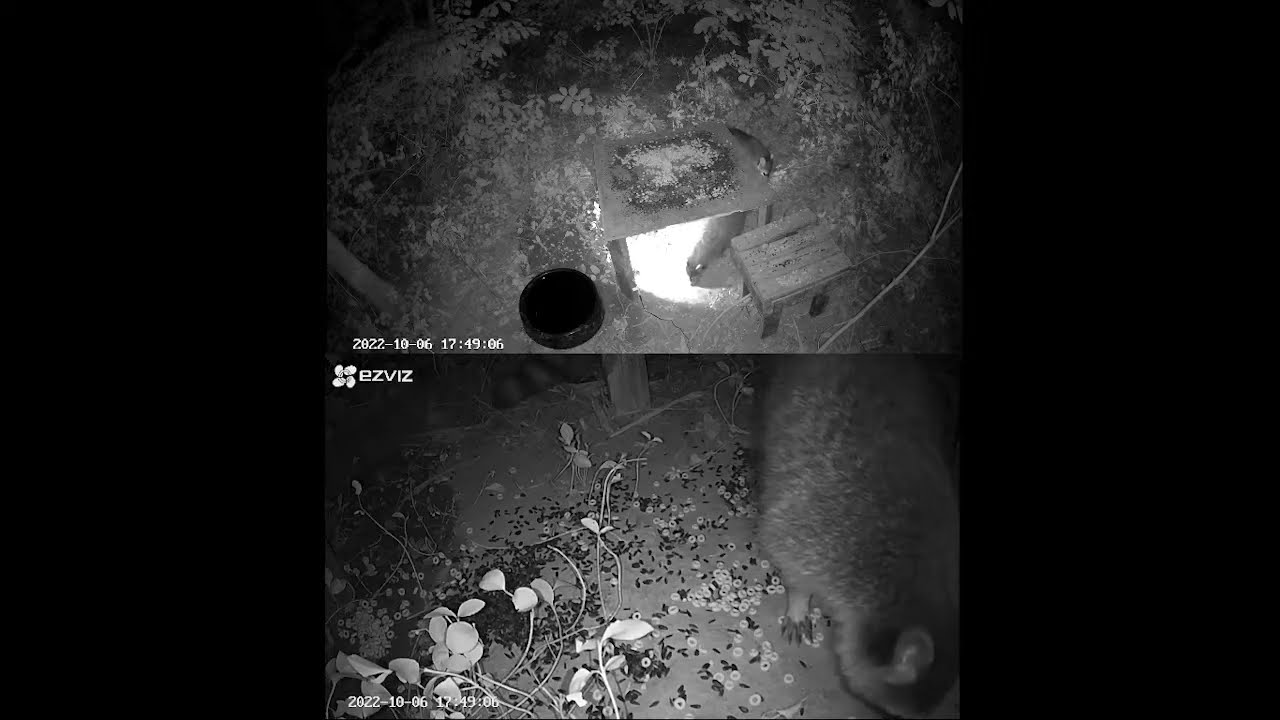This black-and-white double-image appears to be night-vision or low-light footage from a security camera, dated 2020-10-06 at 17:49:06. The top image captures a scene with leaves and a possible den area, featuring what might be a wooden bench or table and a dark circular dish to the left, dimly lit under a small ledge. In the bottom image, an animal, possibly a raccoon, opossum, or fox, is partially visible in the bottom right corner, with its head down. The scene also shows a surface strewn with Cheerios and dead weeds, and there's a noticeable text 'E-Z-V-I-Z' in the upper corner of this image.